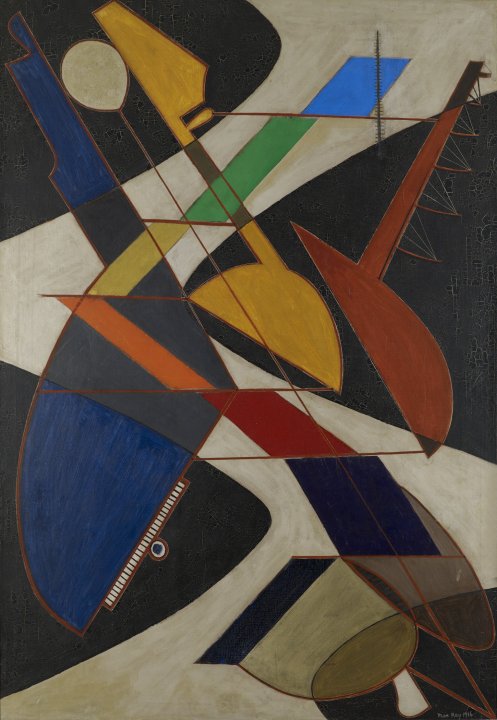This captivating artwork, reminiscent of Pablo Picasso's eclectic style, features a striking collage of black and white interspersed with pops of vivid color. On the right side of the image, a fragmented shape hints at the top part of a string instrument. Interwoven within the abstract composition are splashes of blue, yellow, red, and green, creating a dynamic array of angles and shapes. Among them, a small blue section at the right evokes the appearance of piano keys or perhaps elements of a banjo. At the bottom left, there's an abstract representation that subtly suggests the strings of a violin. The piece as a whole is a vibrant and chaotic exploration of line and form, engaging the viewer in its complexity.